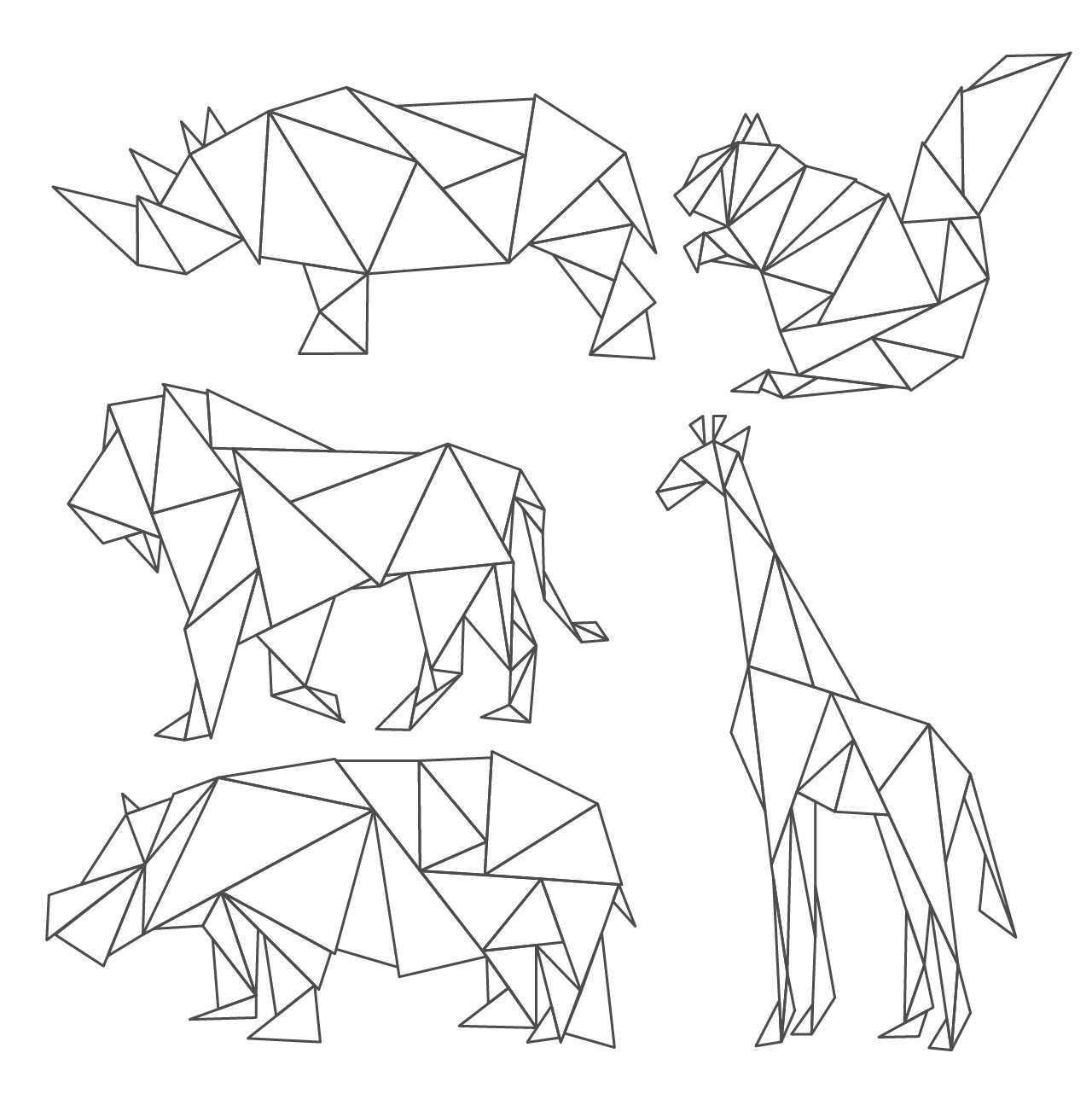The black-and-white image displays intricately detailed polygonal drawings of five animals on a white background, utilizing a combination of variously oriented, shaped, and sized triangles. In the top left corner, there's a rhinoceros facing left, characterized by its distinct horns. To the right, in the top right corner, a squirrel with its tail upraised and its four paws near its mouth stands out as the only non-zoo animal depicted. Centrally located on the left is a lion walking to the left, with its right leg slightly bent. Directly below the lion, in the lower left corner, is a hippopotamus facing left. Meanwhile, occupying the lower right and mid area, is a towering giraffe, also facing left, complete with the long neck and legs typical of its species. The drawings, made with black pencil or line art, emphasize geometric shapes, giving the image a tangram-like quality.